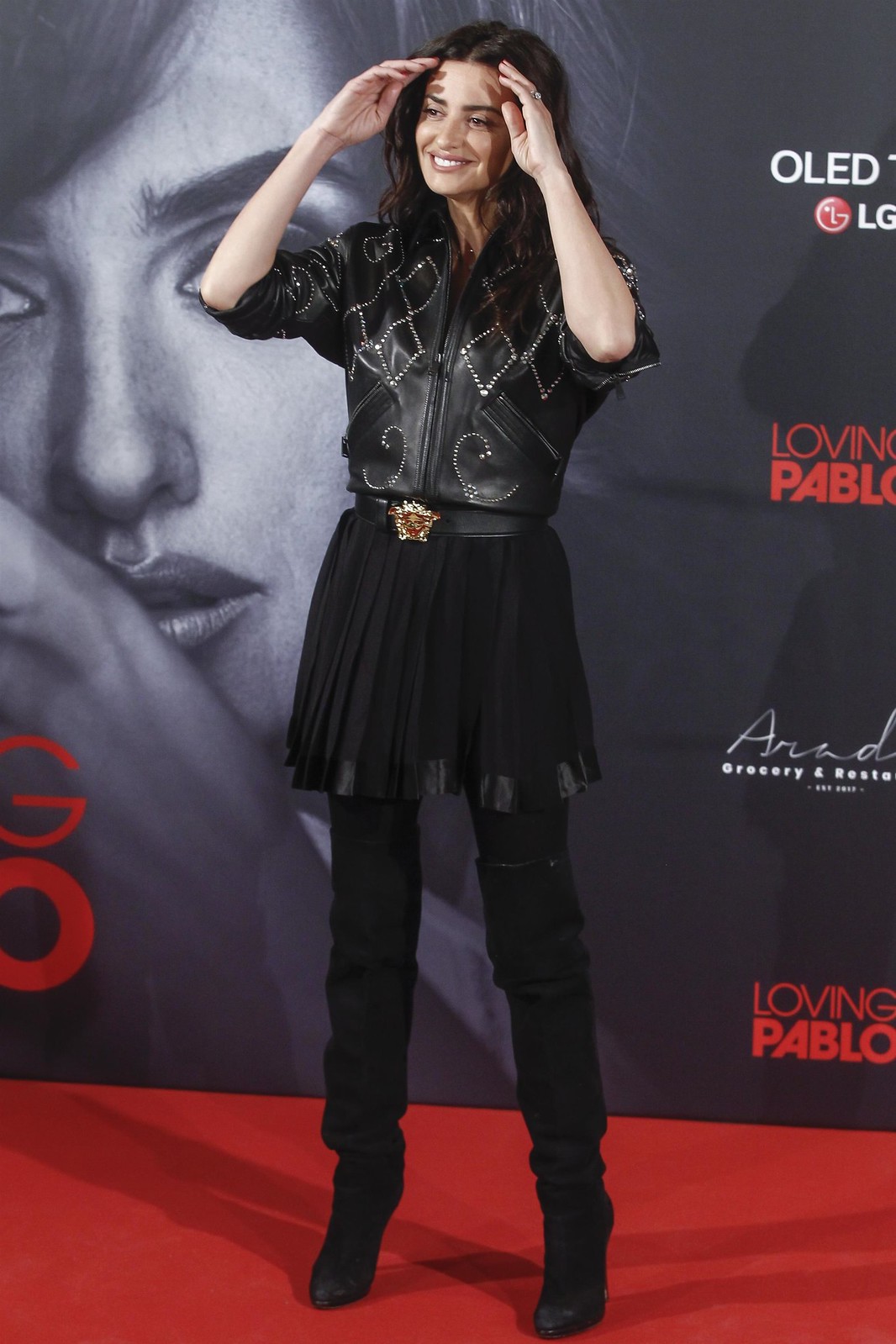The image is a detailed photograph likely taken at a red carpet event, featuring a woman prominently in the center. The woman, posing for the photograph with a smile, is looking directly forward while having her hands raised near her hairline as if shielding her eyes. She is dressed in a striking ensemble consisting of a black frilly skirt and thigh-high black boots. She sports a black leather jacket adorned with a diamond-encrusted pattern, zipped up, and a belt that appears to be made of some type of jewelry at the front. Her hair is black, and she stands confidently on a red carpet, casting a shadow to the left.

Behind her is a partially visible poster featuring an image of a woman in a grayscale filter. The poster includes text that is mostly obscured but notably displays the words "OLED" and "LG" at the top. Below, in red letters, it says "Loving Pablo," repeating at the bottom. Another set of partially visible text in white reads "grocery and resta." The scene captures a blend of glamorous attire and the buzzing ambiance typical of a red carpet event.